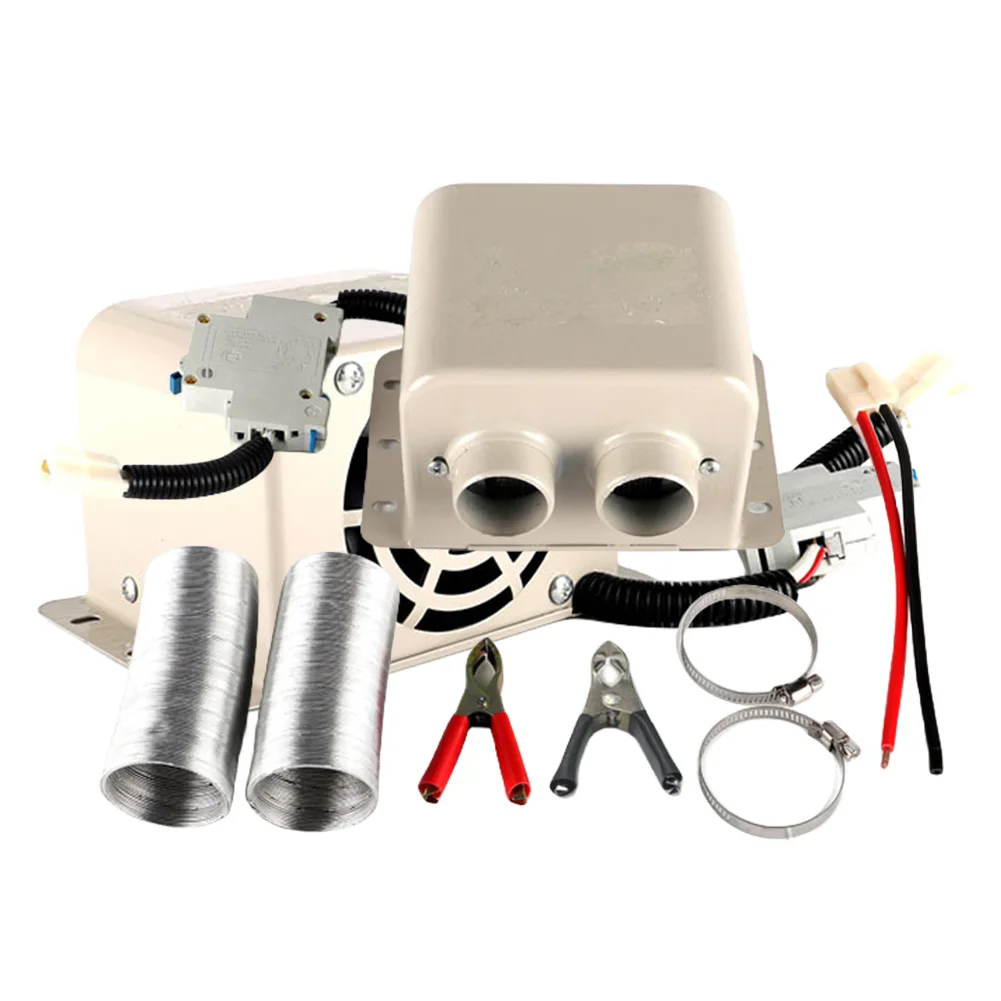The image showcases an array of electrical components and tools laid out on a white background for a product display. Central to the image is a large white metallic box with two circular openings and a series of vents, suggesting it houses a fan or cooling mechanism. Attached to the box is a black pipe with an additional gray box connected to it. Flanking this are two aluminum-like, metallic foil cylinders designed to be expanded, each equipped with adjustable rings for securing attachments.

In addition to the main equipment, the scene includes various tools and wires. Among these are a pair of connectors, one red and one gray, alongside some unclad, cylindrical silver wires. Coated wires, predominantly black and red, are also visible, matching the color scheme of the tools present, which consist of pliers and a wire stripper. The consistent color palette reinforces the cohesive nature of the toolset and equipment, though their specific application remains ambiguous. Overall, it appears to be a comprehensive kit for electrical work involving cooling or exhaust systems.